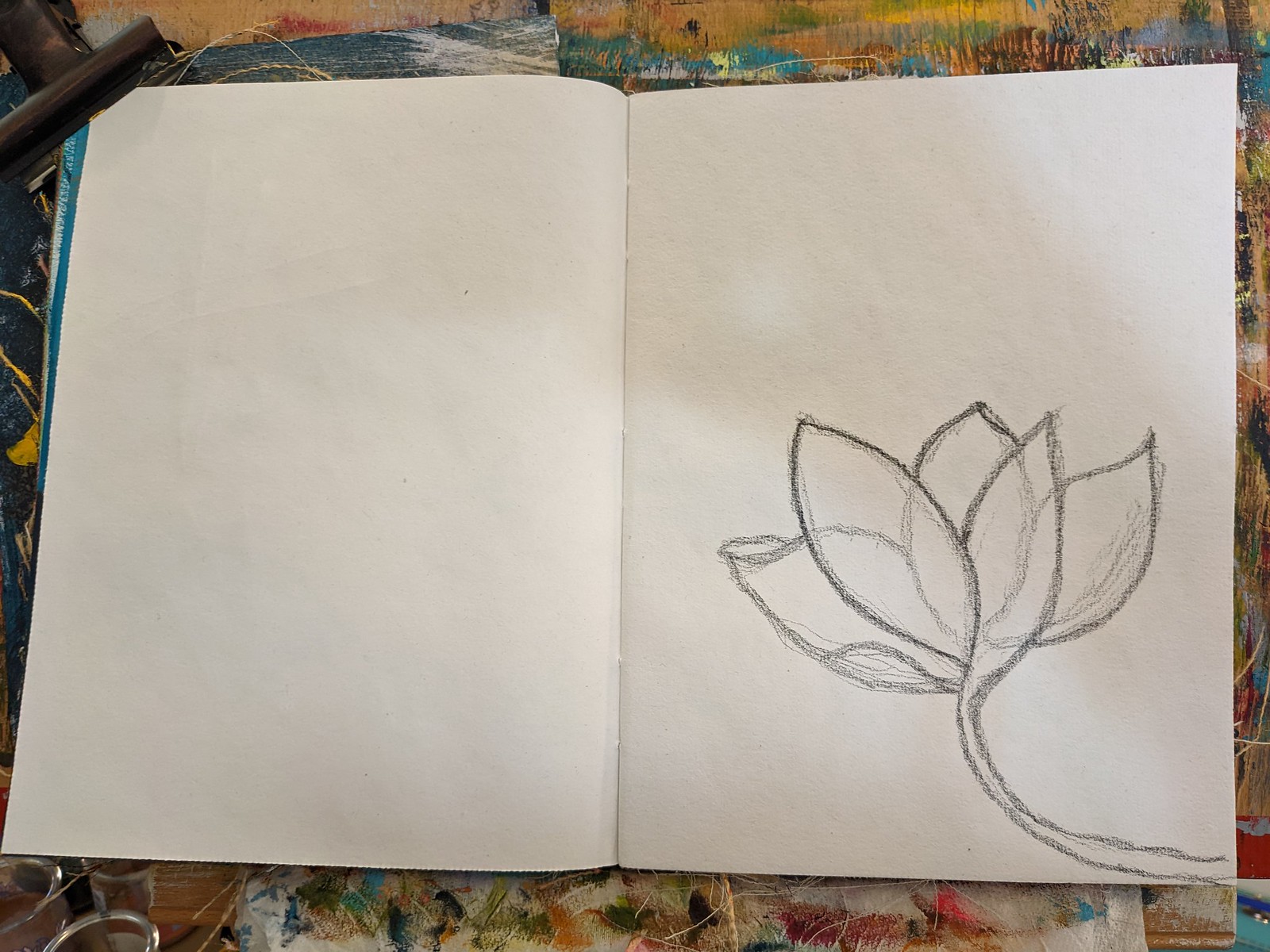This detailed color photograph shows an open sketchbook centered prominently in the image. The sketchbook is positioned on a surface with paint markings, which suggests a well-used art desk. At the top left corner, a binder clip is visible, holding the pages open. The left page of the sketchbook is entirely blank, while the right page features a pencil drawing of a flower, likely a lotus or possibly an unfinished rose. The flower is depicted in side profile with five distinct petals and a center that's partially obscured by the angle of the drawing. A curved stem emerges from the bottom right corner of the page, extending upward to connect to the flower. There is no color in the illustration—only dark pencil lines define the flower and its structure. The image captures the peaceful, creative moment of the artist's workspace, highlighting the blend of simplicity and potential in an unfinished piece of art.